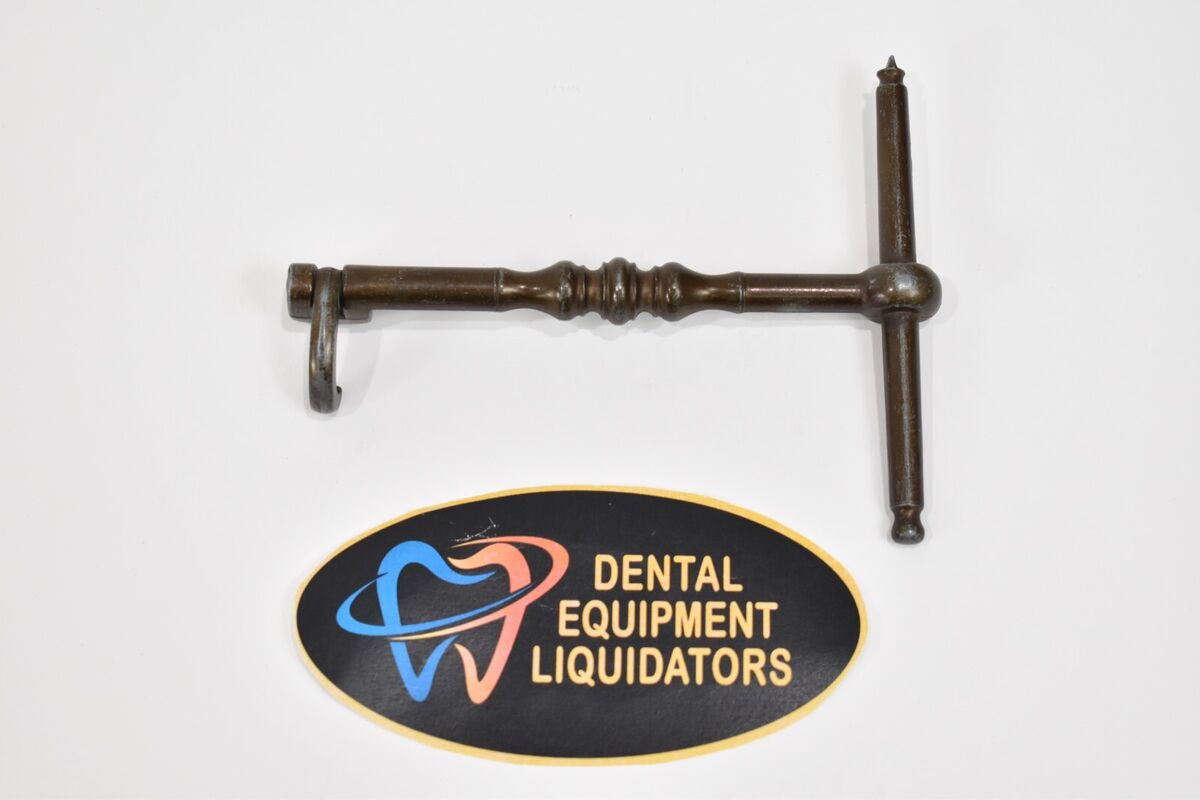The image features a color photograph with a white background. Central to the composition is an antique, dark bronze metal implement resembling a sideways T-shape. It has a long shaft with a pointed tip on one end and a ball-peen knob on the other, some grip-enhancing notches in the middle, and a hook-like extension on the left. The tool's design includes a handle to the right, a shaft with knobs, and a swivel connection. Below this implement is an oval black sign with a gold outline and the text "Dental Equipment Liquidators" in light yellow. The sign also displays a stylized tooth, depicted in blue and pink, with a blue and pink swirl encircling it. The sign appears unattached and rests against the white background. The overall impression is that this could be an old, possibly antique dental tool, situated above branding for a dental equipment liquidator.